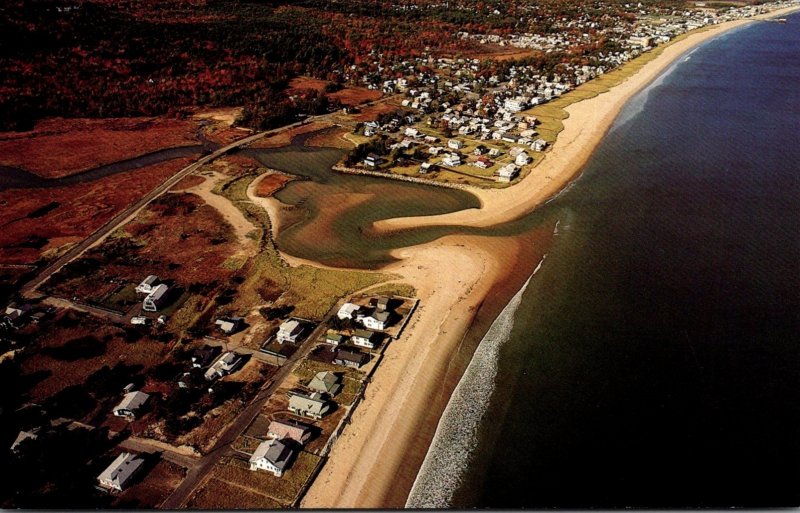This aerial photograph taken from an aircraft depicts a coastline stretching horizontally across the image. On the right side, a very dark blue ocean meets a sandy beach that runs along the entire shoreline, with surf visibly approaching the land. The left side of the image features a mix of agricultural areas, with brown and green cultivated fields, patches of flat land, and some mustard-green vegetation. 

In the middle of the photo, behind the beach, there are clusters of whitish-gray houses and buildings. This central area is less densely populated compared to the upper part of the image, which shows more concentrated housing and a road cutting through the landscape. The road extends along both sides of the shoreline, curving off to the upper right where the image becomes brighter.

Overall, the photograph presents a mixture of sandy, urban, and rural landscapes, with notable dark sections on the upper left and bottom left of the image, highlighting the gradient of density and color. The shoreline also has an inlet further enhancing the scene’s intricate details.